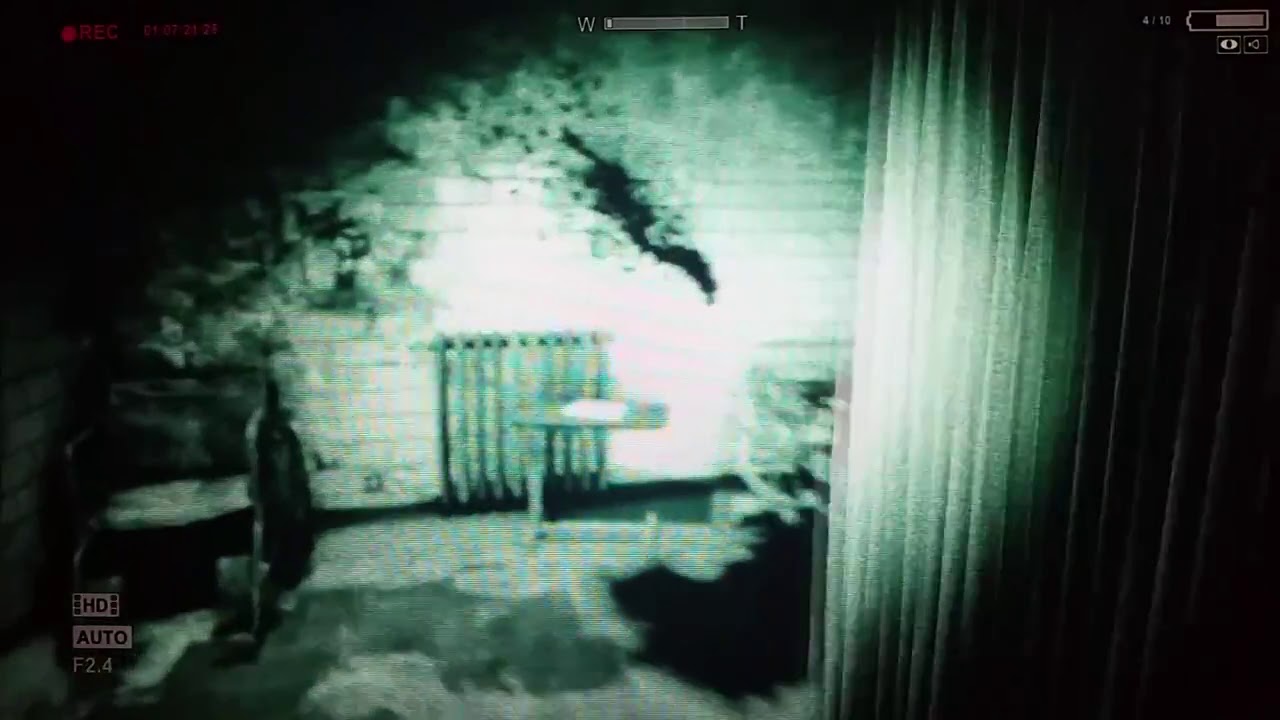This black-and-white photograph, tinged with a dark teal blue or green hue, reveals a dimly-lit, neglected room that exudes a sense of eeriness and decay. The white brick walls in the background are marred with stains and partially obscured by a disheveled curtain extending over about a third of the right side of the image. An old radiator, firmly attached to the wall, hints at the room's age and lack of maintenance. To the left, a weathered, broken-down wheelchair sits abandoned, its dilapidated state adding to the atmosphere of desolation. Scattered objects and dark stains mark the floor, contributing to the room's chaotic appearance. In the middle, a small bedside table rests against the wall, overshadowed by the decaying environment. Barely perceptible, there may be a bed frame near the table, adding to the room's cluttered and distressed look. Faint, illegible text on the bottom left edge hints at some forgotten context, while a hazy aura envelops the scene, amplifying the room's haunting ambiance.